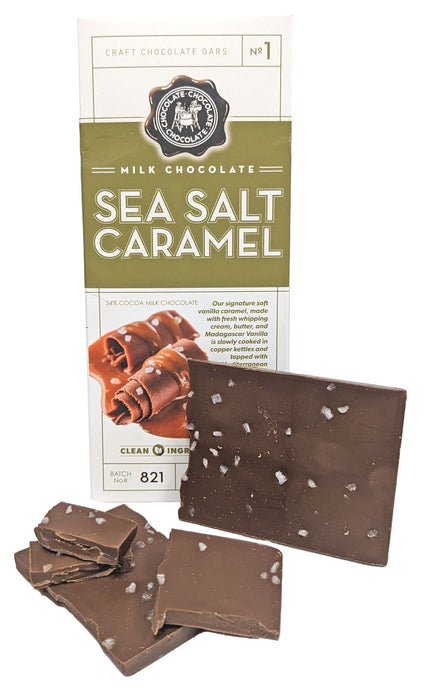The image depicts a sea salt caramel chocolate bar with its packaging prominently behind it. The chocolate bar, positioned in the foreground, is broken into several pieces: four smaller pieces in the lower left corner and a larger piece leaning against the packaging. The chocolate itself is a rich brown color, dotted with large flecks of white sea salt, giving it a distinctive, textured appearance. The packaging in the background is primarily white with a central olive-green rectangle that reads "Milk Chocolate, Sea Salt Caramel" in white font. Above the green rectangle, a circular logo states "Chocolate Chocolate Chocolate." At the very top of the packaging, it says "Craft Chocolate Bars No. 1," while the bottom left includes the batch number "821" in black. Additionally, the packaging features an image of the chocolate and a partially visible description extolling the virtues of their soft vanilla caramel made with fresh whipping cream, butter, and Madagascar vanilla, cooked in copper kettles. The overall image is set against a clean, white background with bright and clear lighting, highlighting the details of both the chocolate and its packaging.